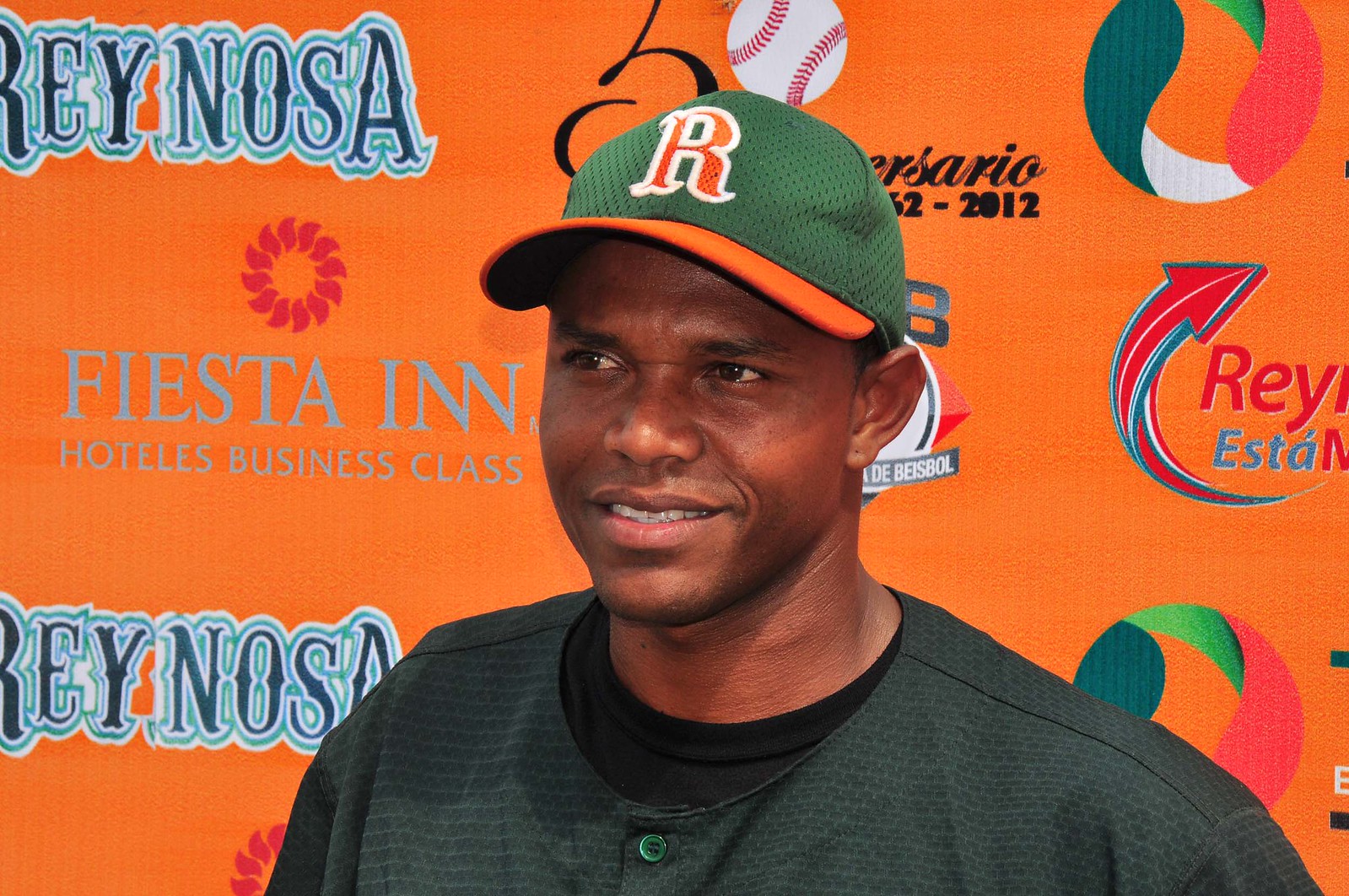This is a close-up, colored photograph of a dark-skinned male, who appears to be a sports player. He is dressed in a dark green sports shirt layered over a black t-shirt, accompanied by a green and orange baseball cap with an orange 'R' prominently displayed on the front. The cap has an orange brim and the green fabric contrasts sharply against his clean-shaven face and brown eyes. He is looking slightly to the left, smiling gently as if recounting a pleasant memory. Behind him is a vibrant orange backdrop adorned with various logos and text. Notably, there is the word "Reynosa" in blue letters outlined in light blue, "Fiesta Inn Hotels Business Class," and phrases in Spanish like "Esta De Beisbol." Additional illustrated elements include a baseball and a round, colorful circle near his shoulder, as well as an image resembling a bright sun with an orange center and a red rim, enhancing the strong, warm tones of the overall composition.